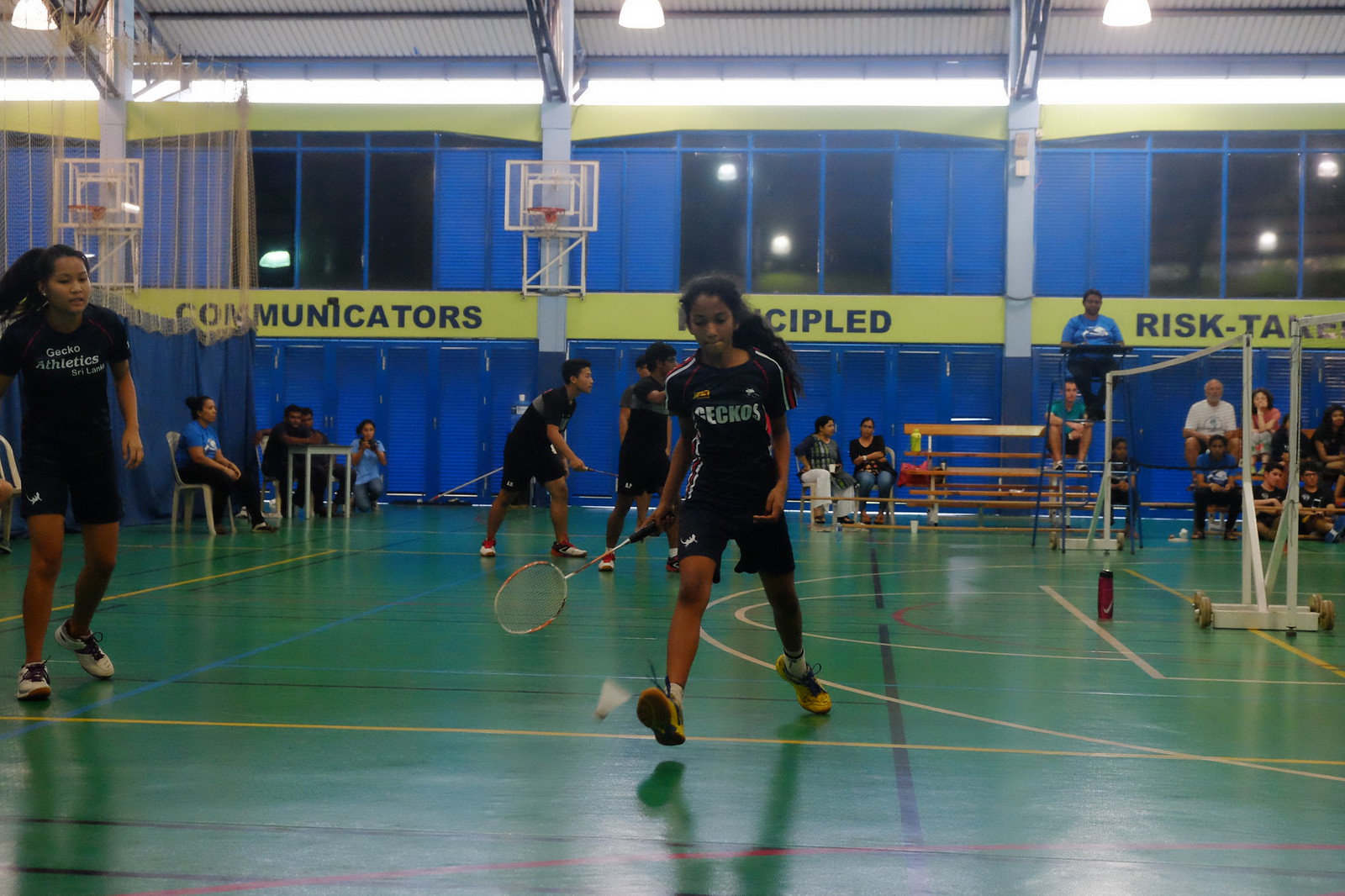In this detailed sports photograph, a young girl is captured mid-action inside a gymnasium, participating in what appears to be a mixed-gender badminton game. The gym features green flooring and visible basketball nets, indicative of a multi-sport facility. The focal point is the young girl, energetically moving towards the camera. She is dressed in a black uniform consisting of black shorts and a black jersey top, emblazoned with the team name "Geckos." Her long, full curly ponytail is dynamic and adds to the sense of movement. In her right hand, which appears to be on the left side of the photo, she holds a badminton racket, aiming to hit the birdie, or shuttlecock, suspended in the air. 

Scattered around the gym, other children—both girls and boys—are also engaged in the game. Notably, another teammate is slightly in the background to the girl's right (left in the image), wearing a black t-shirt with "Gecko Athletics," which differentiates from the primary jersey. This teammate seems poised, possibly contemplating making a move for the birdie, adding a layer of strategy to the scene. The photograph vividly captures the intensity and spirit of youth sports within this communal, indoor arena.